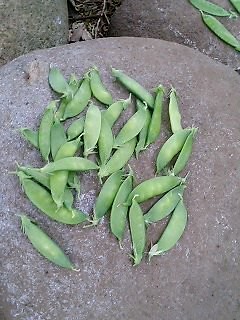The image depicts a zoomed-in, top-down view of a large, round, dark gray rock with a collection of freshly picked green pea pods scattered on its surface. The pea pods, roughly three to four inches long and a light to medium shade of green, form a loose circle and overlap in places. Approximately 20 to 25 pods can be seen on this main rock, many with small white strings emerging from the tips where they were picked, and accompanied by some loose greenery. These pods are plump, indicating the presence of peas inside, akin to sugar snap peas. In the upper right and left corners of the image, background rocks of varying dark gray hues are visible, each hosting a few additional pea pods. The upper rocks are interconnected by scattered sticks or mulch, adding natural texture to the scene.